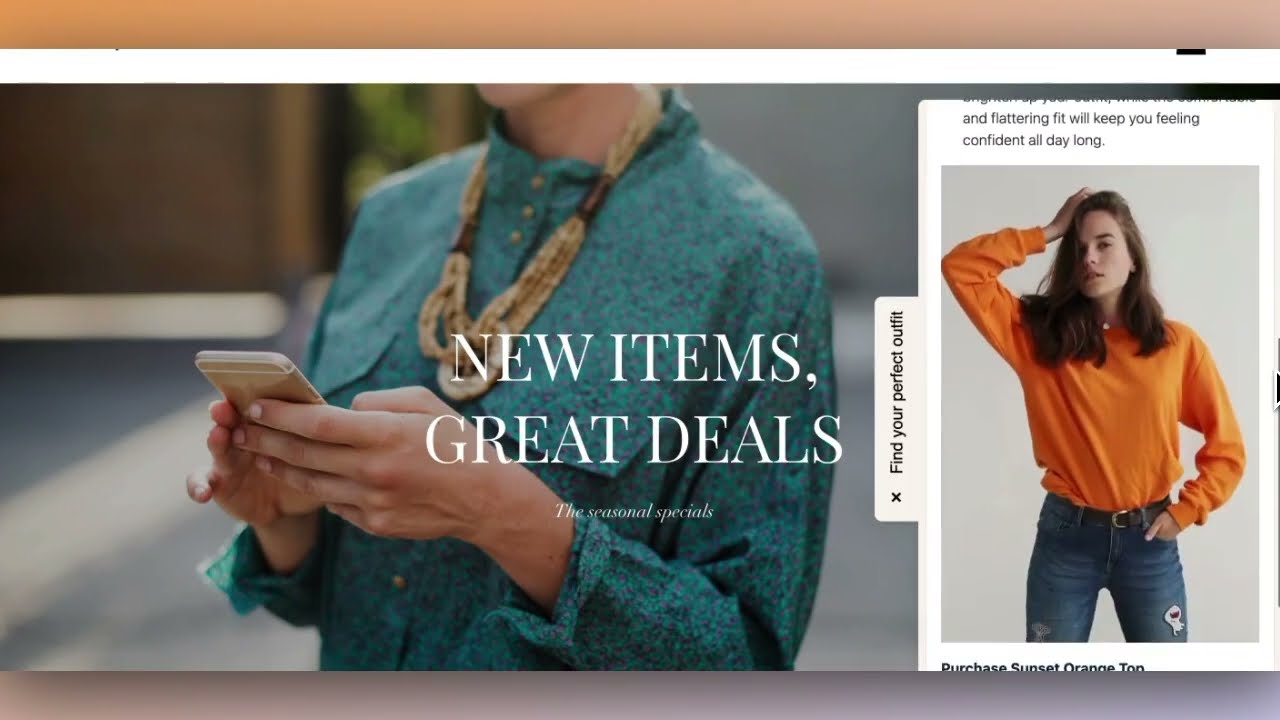This image is a screenshot from an unspecified e-commerce website, with the header partially cut off, obscuring the retailer's name. The visible part of the header is bronze on the left and a light purplish-gray on the right. Central to the image is a large photo focusing on a woman's upper torso. She is a white woman with only the bottom of her chin and her neck visible. She is dressed in a delicate, silk-like blouse in shades of green and blue, which has a high neckline with three gold buttons. Around her neck, she wears a multi-strand necklace of light brown seed beads, and she holds a smartphone in both hands, with only the top back of the device visible. Overlaid on this photo in white font are the words "New Items, Great Deals," with "The Seasonal Specials" written in smaller font beneath it.

To the right of this central image is another photo, showing a full-body shot from head to mid-thigh of a young white woman, likely in her mid to late 20s. She has dark brown hair that falls just below her shoulders. She is dressed in an orange long-sleeve shirt, blue skinny jeans, and a brown belt.